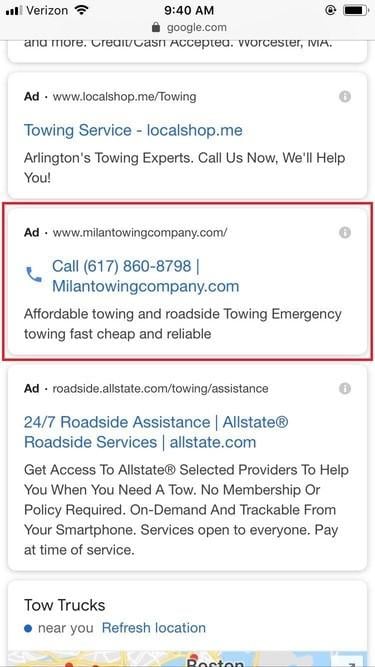This screenshot displays a series of Google ads organized in a vertical column, each within its own distinct white box. The contents of the ads are as follows:

1. The first ad is from "localshop.me" offering towing services in Arlington.
2. The second ad, highlighted by a red border, is from "Milan Towing Company". It prominently features a contact number, 617-860-8798, alongside the website "milantowingcompany.com".
3. The third ad, from "roadsideallstate.com", advertises 24/7 roadside assistance through Allstate Roadside Services.
4. The final ad on the list is titled "Tow Trucks Near You" and includes a partially cut-off map, seemingly depicting the Boston area.

At the top of the screen, the status bar indicates the time as 9:40 AM, alongside a lock icon signifying a secure connection to google.com, and a battery icon in the top right corner. Each ad box features a grayed-out information icon at its top right. The overall webpage and the individual ad boxes maintain a white background.